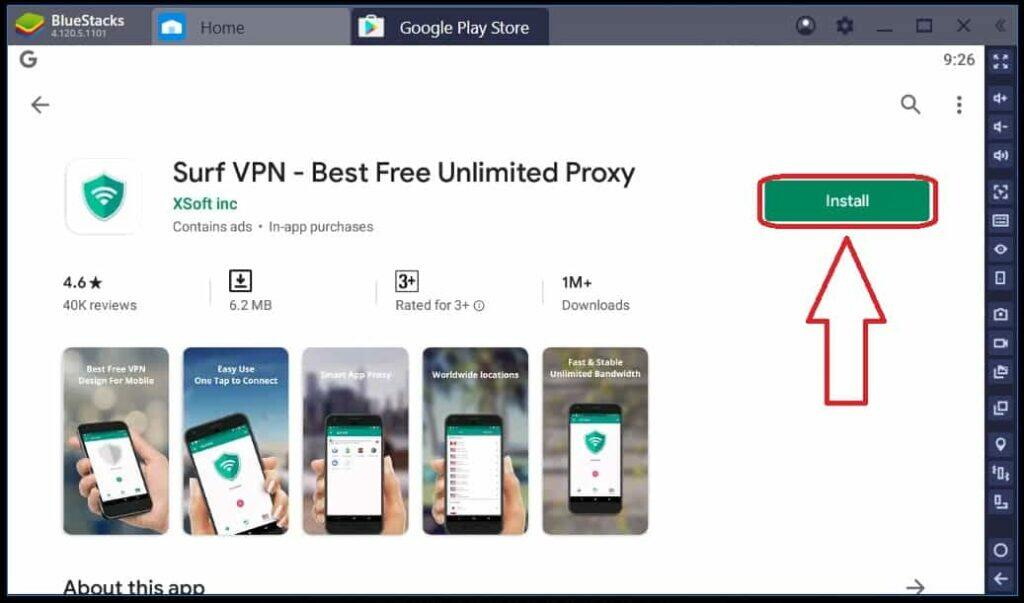The image appears to be a screenshot captured from a computer, displaying an open BlueStacks application. The image showcases three tabs at the top: "BlueStacks," "Home," and "Google Play Store," with the latter active. The top section of the screen features a grayed-out rectangular bar and includes the Google logo at the top left, while a digital clock in the top right corner indicates the time as 9:26. 

Directly underneath the Google logo, a back arrow and a search icon are visible, followed by the text "Surf VPN - Best Free Unlimited Proxy" and "XSoft Inc." Below this, a note states the app contains ads and in-app purchases. A prominent green 'Install' button is positioned to the right, highlighted by a red outline and an upward-pointing arrow beneath it. 

The central section of the screen displays five thumbnail images, each showing different features and pages of the Surf VPN app. Beneath these images, the text "About This App" is visible. On the right side of the window, a sidebar contains a collection of quick links related to Google services, though their functions are not specified. 

The details provided up to this point create a comprehensive description of the screenshot, encapsulating its elements and layout.